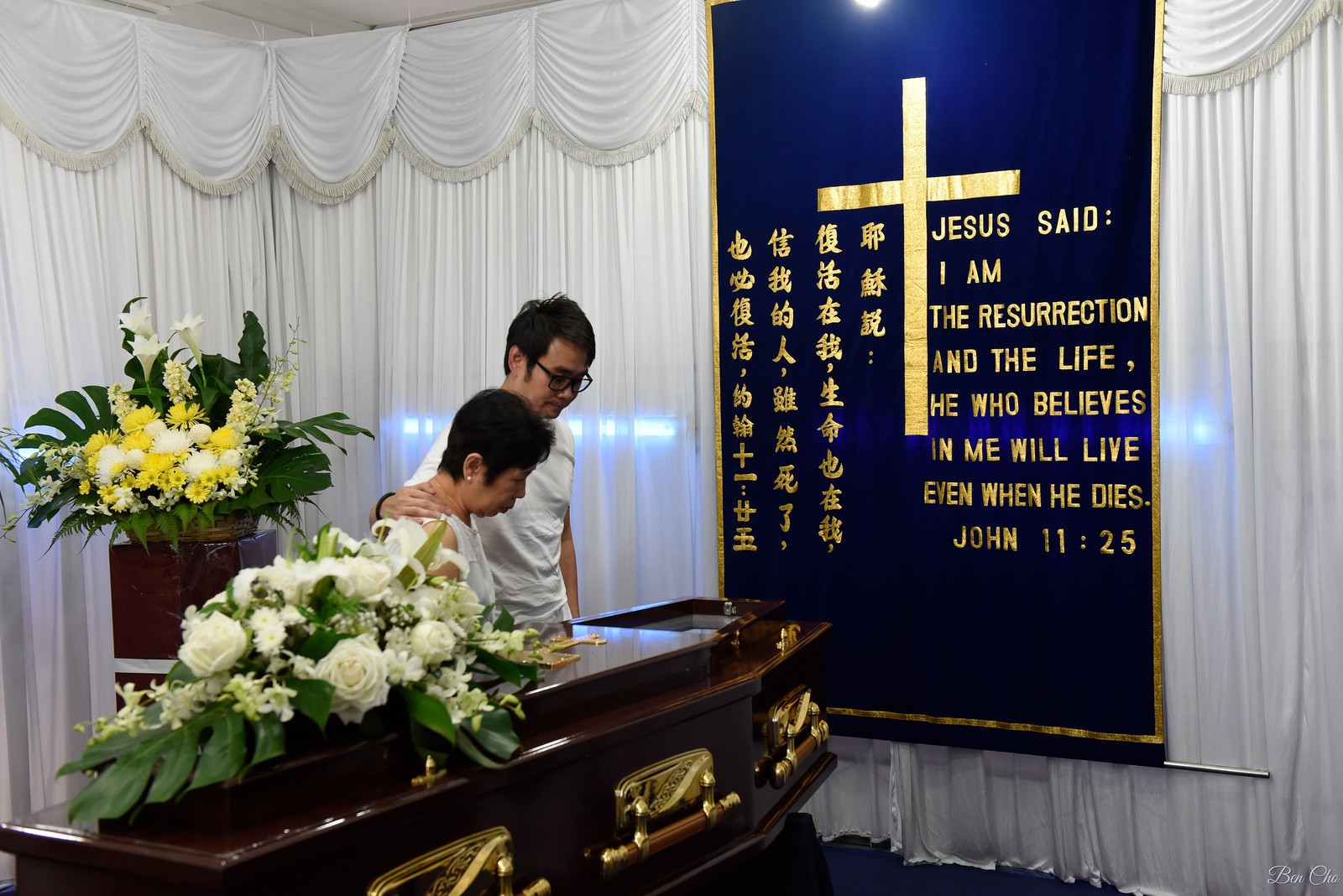This horizontal-rectangular color photograph captures a solemn moment at a funeral home. In the foreground, an ornate open casket is adorned with a beautiful arrangement of white flowers. Standing beside the casket are two individuals, an older Asian woman and a middle-aged Asian man, who are looking down into it. The man has his right arm gently resting around the woman's shoulders, offering comfort. Behind them, a closed white curtain provides a sense of privacy, with faint car headlights visible through the fabric.

On the right side of the image is a prominent navy blue banner featuring a large gold cross in the center. The banner has gold lettering in both Chinese and English. The English text reads, "Jesus said, I am the resurrection and the life. He who believes in me will live even when he dies," followed by the Bible reference John 11:25. In addition to the flowers on the casket, there are more yellow and white flowers on a pedestal behind the pair, enhancing the decor of the space. The combination of muted colors and the solemn expressions of the individuals convey a poignant and respectful atmosphere.